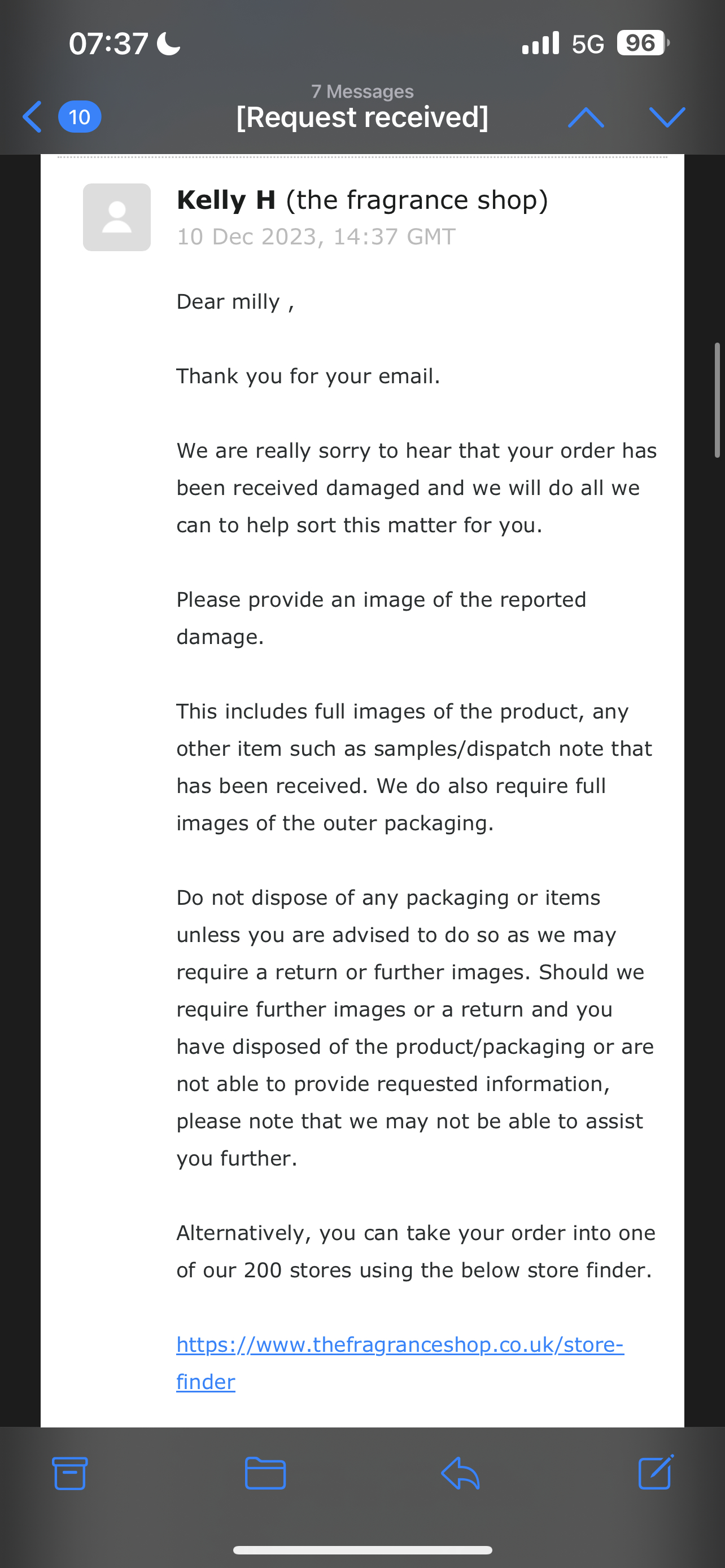Screenshot of a smartphone screen taken on 10 December 2023 at 14:37 GMT, showing a battery level of 96% and a notification for seven message requests. The open message is from Kelly H at The Fragrance Shop, addressing a customer named Millie. The message reads:

"Dear Millie,

Thank you for your email. We're really sorry to hear that your order was received damaged, and we will do all we can to help sort this matter for you. Please provide an image of the reported damage. This includes full images of the product, any other items such as samples, and the dispatch note that you received. We also require full images of the outer packaging. Do not dispose of any packaging or items unless advised to do so, as we may need further images or a return.

Should we require further images or a return and you have disposed of the product/packaging, or are unable to provide the requested information, please note that we may not be able to assist you further. Alternatively, you can take your order into one of our 300 stores using the store finder below."

There is a link to the store finder at the end of the message.